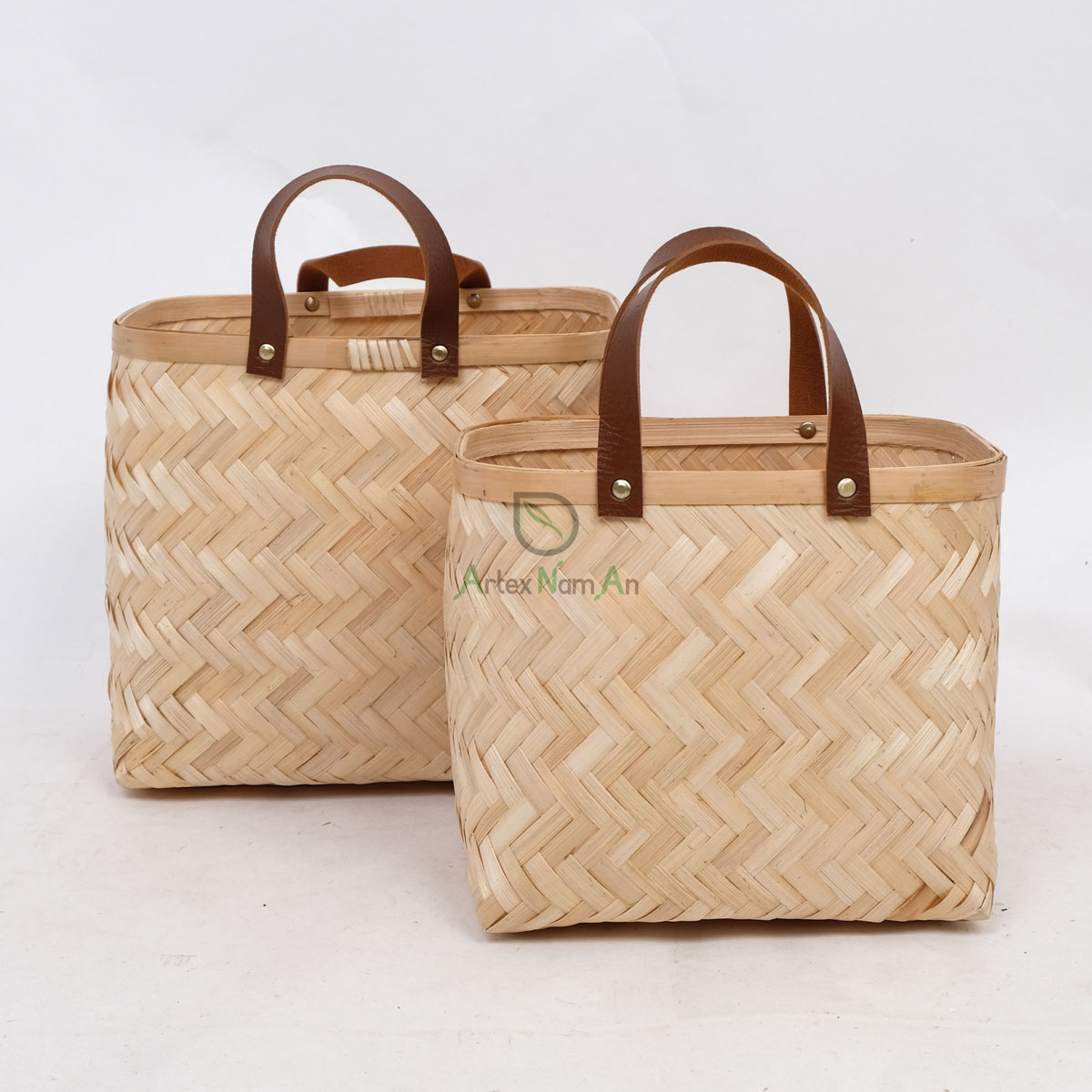The photograph features two woven tote bags, one slightly larger and positioned behind the other, creating a staggered composition. Crafted from a wood-like fiber, the totes exhibit an intricate chevron or zigzag pattern in a natural tan hue. Each tote is adorned with a light brown band at the top, and dark brown leather handles secured with metal rivets. This fastening detail contributes to the bags' sturdy appearance. Overlaying the image, in the center, is the text "Artex Nam Ann" with the first letters of each word highlighted in green and the remaining letters in brown or gray. Accompanying the text is a symbol resembling a leaf incorporated into a pointed circle, suggesting a theme of sustainability. The clean, white background and professional lighting make the photograph appear as though it could be part of a catalog or advertisement, emphasizing the detailed craftsmanship of the totes.